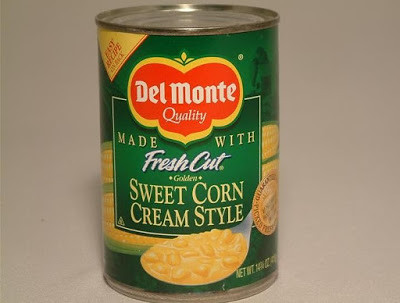The image features a can of Del Monte brand sweet corn cream style with a distinctive label. The background is medium gray, appearing lighter at the bottom due to the lighting. The can itself has a silver top, typical for can openers. The label is green with a yellow triangle in the upper left corner. There's a prominent red and yellow emblem reading "Del Monte Quality." Below, a green rectangular section states "Made with fresh cut sweet corn cream style" in light green text on a darker green background. A graphic of a silver spoon holding creamy corn is displayed, showcasing the product. There is also a gold circle on the right side that might be an award or additional information, while the net weight is listed at the bottom, partially visible, possibly reading 14 ounces. The top of the can mentions an "easy recipe" with instructions on the back.